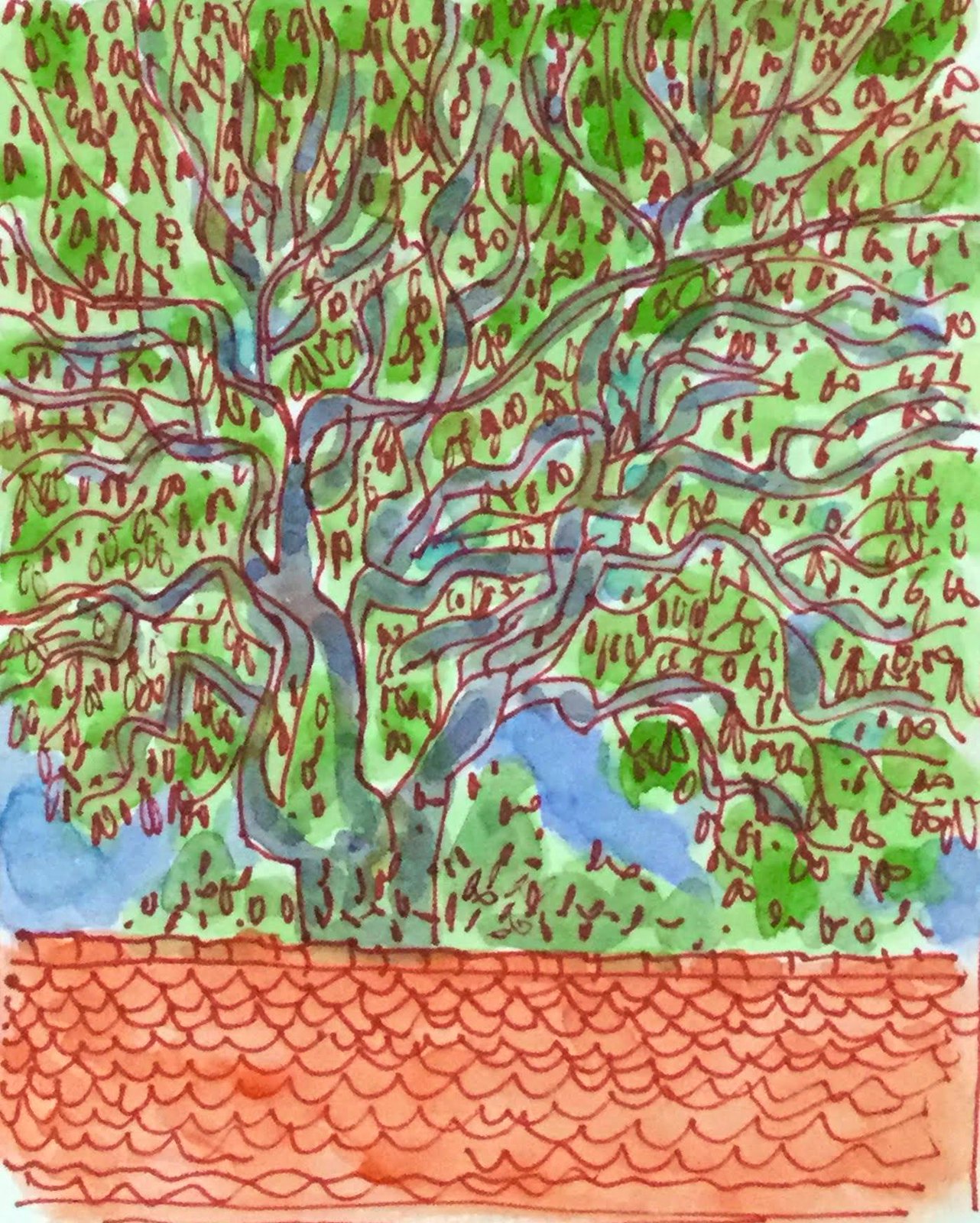The artwork is a watercolor painting primarily depicting a large tree with bluish-gray branches and trunk, created with a combination of red pen or marker and blue paint. The tree’s foliage is painted green, with additional red accents that may signify leaves, flowers, or fruit. Surrounding this tree are additional trees, giving a sense of depth and a lush, verdant landscape. The foreground features an intriguing pinkish ground that may suggest rippling water or textured earth; this ground is composed of wavy, pointy lines drawn in red, further enhancing the overall texture. The background offers a peek of blue sky, contrasting notably with the green tones dominating the scene. The painting's composition and color palette might evoke an oriental or Chinese landscape painting, filled with intricate details and natural elements.